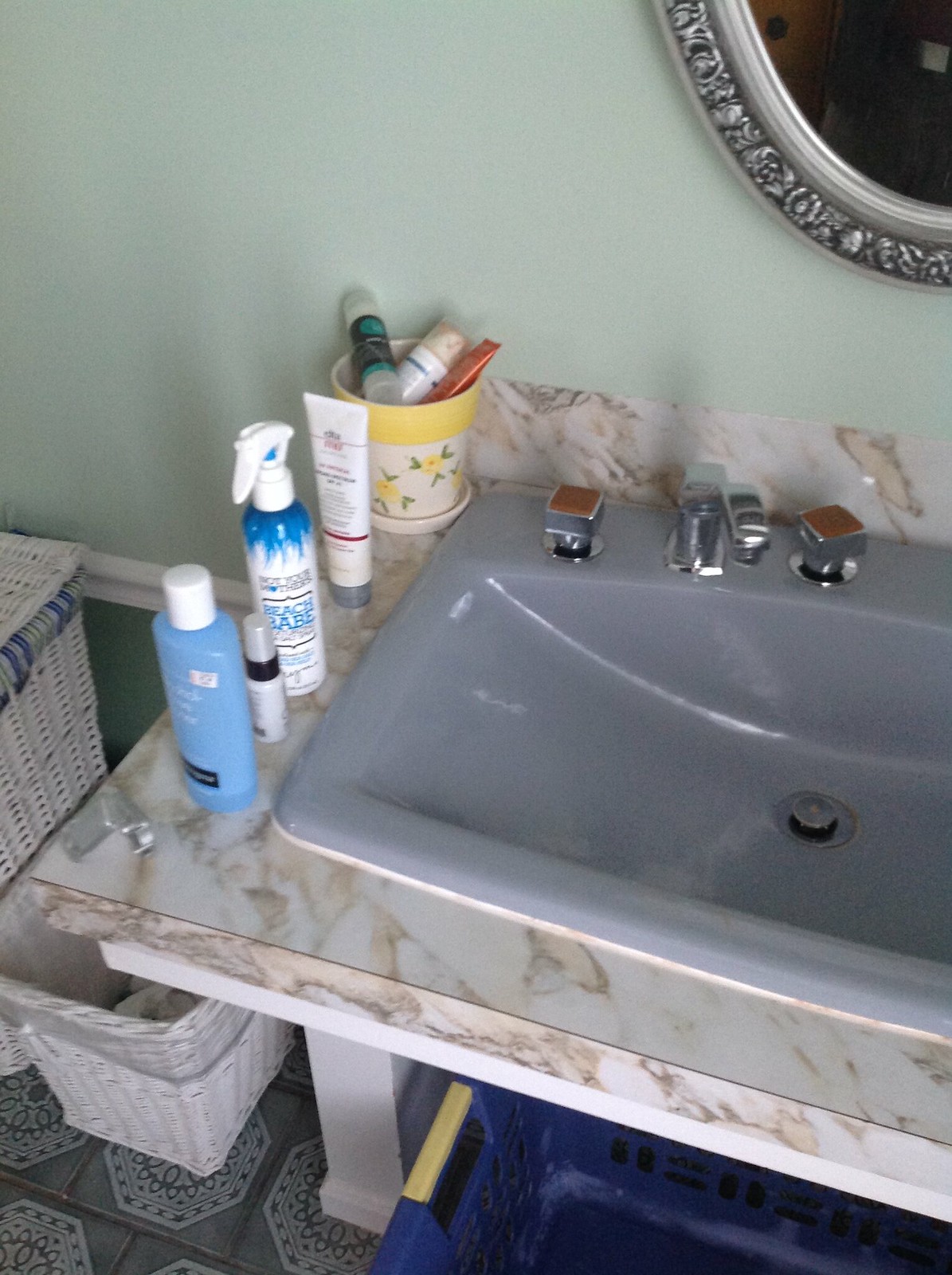In this cozy home bathroom, a light grey-blue sink with two knobs featuring brown or orange tops stands out on a marble-style base, which appears to be wood with a laminate finish. The sink is complemented by a shiny, silver-colored ornate oval mirror that hangs on a mint green wall. The grey tiled floor below has a unique design with light grey octagons accented by dark grey details. At the bottom left, two white storage baskets of different heights rest beside the sink. Underneath, there is a dark blue plastic laundry basket with yellow handles. To the left of the sink, various products, possibly including tanning lotion and skincare items, are neatly arranged. A small plant in a pot also sits to the left, accompanied by smaller products, adding a touch of greenery to the space.